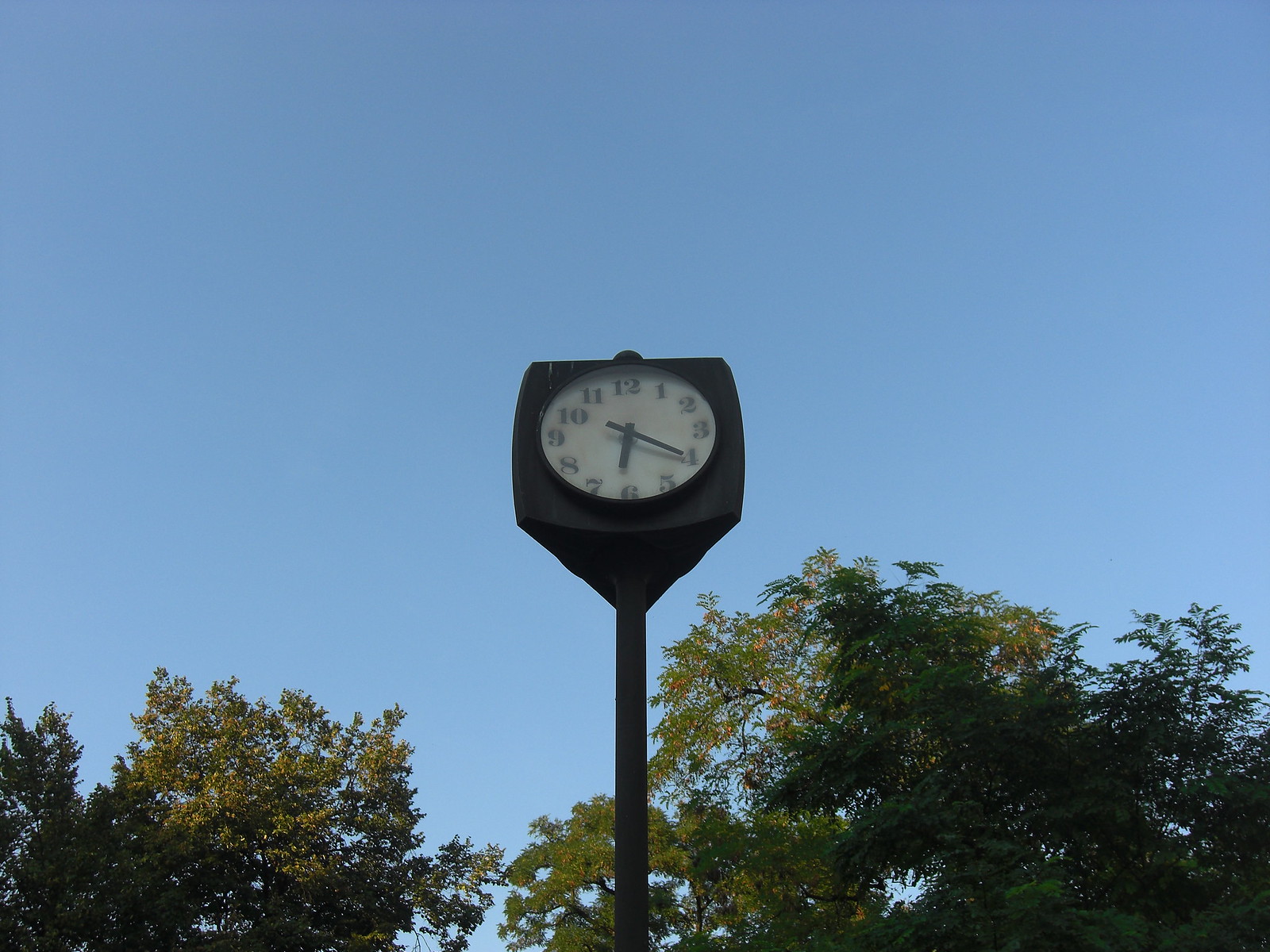The photograph captures a traditional square clock mounted on a tall black metal pole, prominently set against a clear blue sky. The white face of the clock features black numbers and hands, indicating the time as 6:21. The clock appears to have three faces, suggesting its visibility from multiple directions. In the background, two treetops are visible; the left tree is smaller and green, while the larger tree on the right has some yellow foliage, extending from the bottom right corner to the center of the image. The scene evokes a tranquil street setting with an emphasis on the crisp details of the clock and the surrounding natural elements.